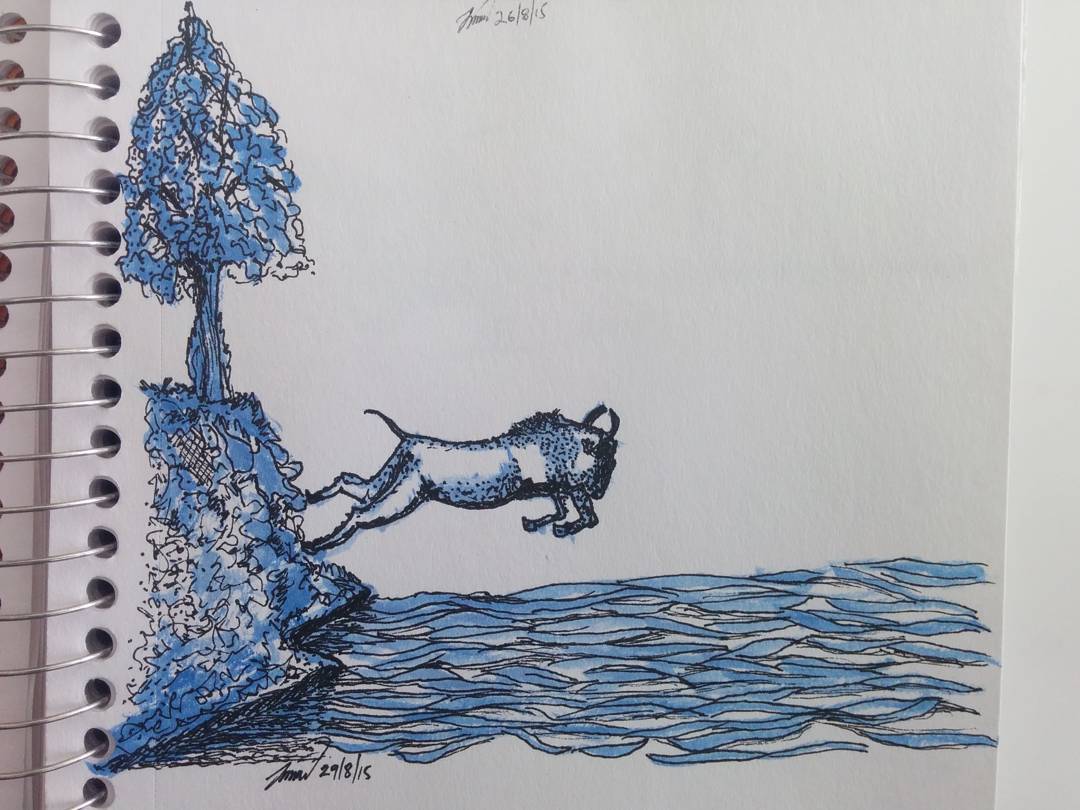This detailed hand-drawn sketch, created with ink and resembling watercolor, is on an off-white spiral-bound notebook positioned on a whiter flat surface. The artwork is signed at the top with an undecipherable name and the date 26/8/15, which likely signifies August 26, 2015. The centerpiece of the sketch is a four-legged, horned animal—possibly a goat—captured in mid-leap, with its back legs still grounded while its front legs and body dive forward toward a blue, ribbon-like representation of water. To the left of the animal, a meticulously detailed blue and black rocky outcrop extends upward, crowned by a tree growing out of its side, enveloping the dynamic scene in a surreal aura. The fluid motion and bold lines of the creature and the surrounding nature elements blend seamlessly, displaying an intricate blend of artistic techniques and surrealistic expression.